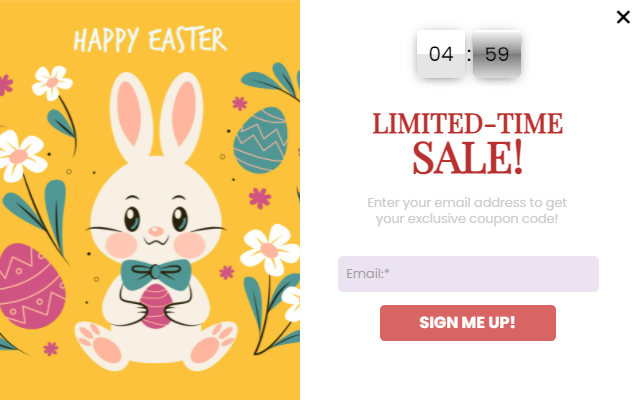Here is the cleaned-up and detailed caption:

"This vibrant Easter-themed card showcases a cheerful holiday design. The background of the card is a bright yellow, adorned with artistic graphics of colored Easter eggs. One egg is blue while the other is turquoise, each embellished with small yellow squiggle lines. The festive greeting 'Happy Easter' is elegantly scripted in white at the top.

At the center of the card, a cute bunny wearing a green bow tie holds a pink egg and gazes directly at the viewer. The bunny also has adorable pink under-toes. To the right, a calendar-style time clock displays '4:59,' and there is a prominent red 'X' marking it with the text 'Limited Times.'

Below, the landing page invites you to 'Enter your email address for your exclusive coupon code.' A lavender-colored input box is highlighted for entering the email address, and a bold red button with white text reads 'Sign Me Up.'

The card is further decorated with three white flowers, two Easter eggs, and small green decorative dots, adding a touch of springtime charm to the overall design."